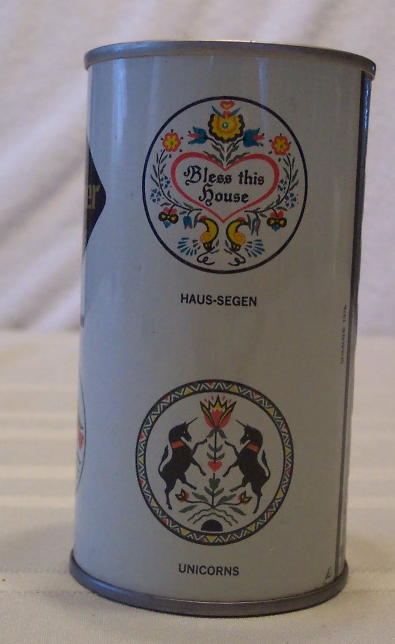A photo depicts a tall, shiny white metal canister resting on a light-colored table with faint horizontal white lines. Behind the canister, a white rippled cloth serves as the backdrop. The canister features two decorative black circles arranged vertically, with elaborate Pennsylvania Dutch designs inside. The top circle showcases a red-outlined heart surrounded by flowers, with the phrase "Bless This House" and a black inscription that reads "Haus Sagan" underneath. The bottom circle contains intricate designs of two black unicorns standing on their hind legs, adorning a central flower motif. Below this circle, the word "Unicorns" is inscribed in black. The canister also has a raw silver metal seam running down its side, and metal rims on both its top and bottom edges.